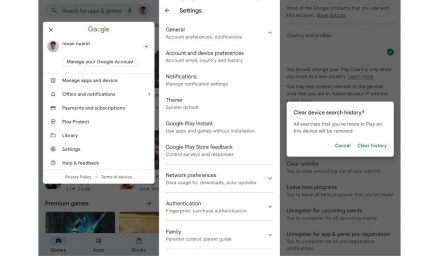The image is a screenshot of the settings page from a Google profile, showcasing the various customization options available to the user. 

In the center, the settings menu is prominently displayed with an arrow pointing to the detailed sections below. These sections include tabs labeled "General," "Account and Device Preferences," "Notifications," "Themes," "Google Play In-Store," "Google Play Share Feedback," "Network Preferences," "Authentication," and "Family," each containing specific descriptions under their respective headings.

To the left of the settings menu, the Google profile details are present. At the top, the unmistakable Google logo, characterized by the colorful font, is visible. Below the logo, there's a profile picture of the user, along with various tabs and options tailored for modifying their personal profile settings.

On the right side of the screenshot, there's a grayed-out, elongated rectangle with a white rectangle inside it containing the text "Clear Device Search History." Beneath this command, it explains that clearing the history will remove all searches made in Google Play, providing options to either "Cancel" or "Clear History."